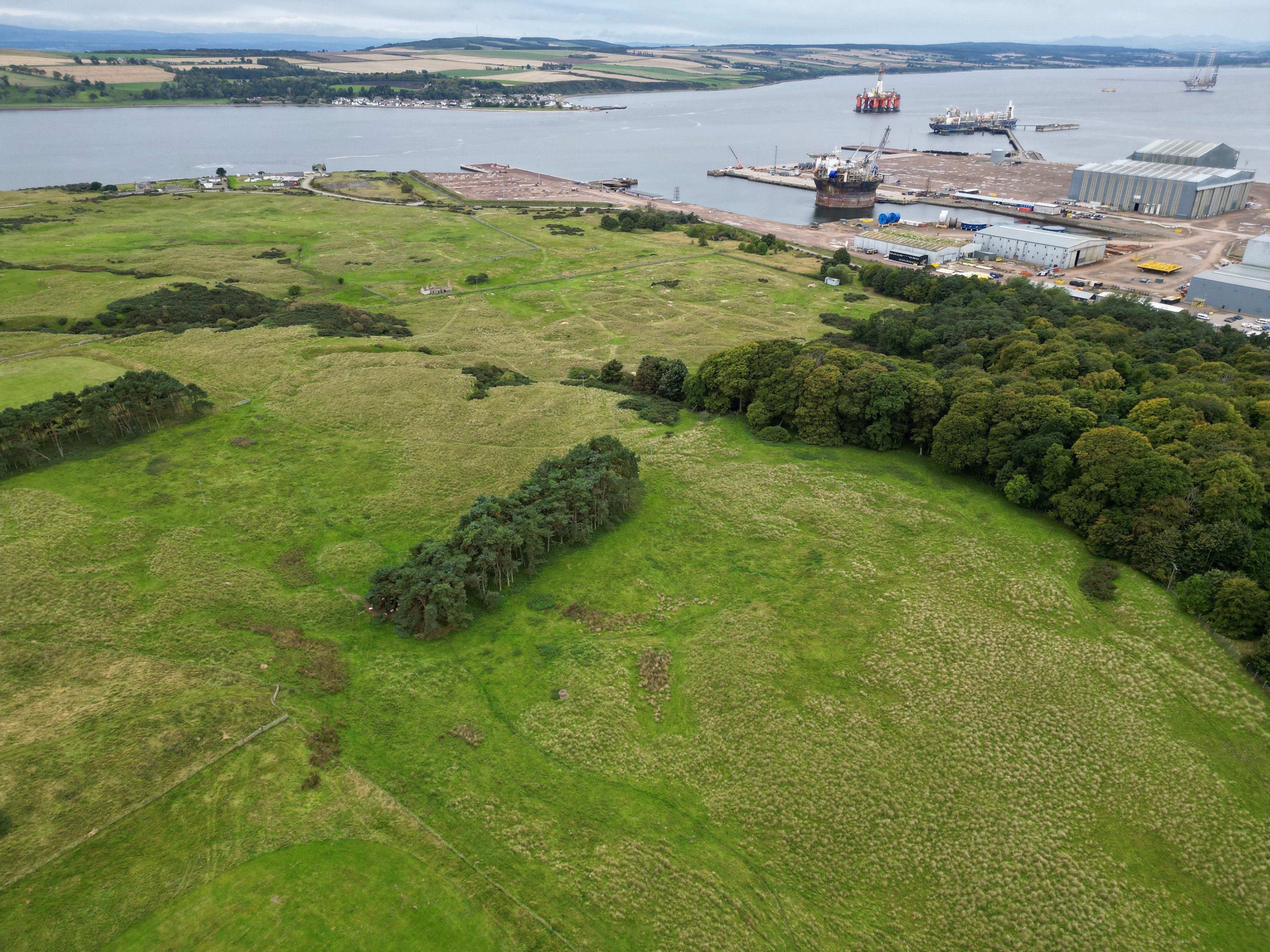This daylight aerial photograph, possibly taken from a drone, captures a high vantage point view of a sprawling green field interspersed with patches of brown, likely indicating the onset of fall. The field features pockets of trees, including a thick forested area and a couple of neatly aligned rows of trees, giving the terrain a hilly appearance as it stretches towards a substantial body of water in the top portion of the image. This waterway—potentially a river or inlet—is home to large ships, including cargo vessels and what resembles a permanent platform structure.

On the right, bordering the water, a port facility stands with visible white and pale blue warehouses and a possible crane structure. The docks are busy with trucks and other vehicles moving about. Opposite the river, the land transitions into another cultivated field with brown patches, suggesting agricultural activity. The overall scene, likely reminiscent of the Midwest United States, is overcast, hinting at recent or impending rain.